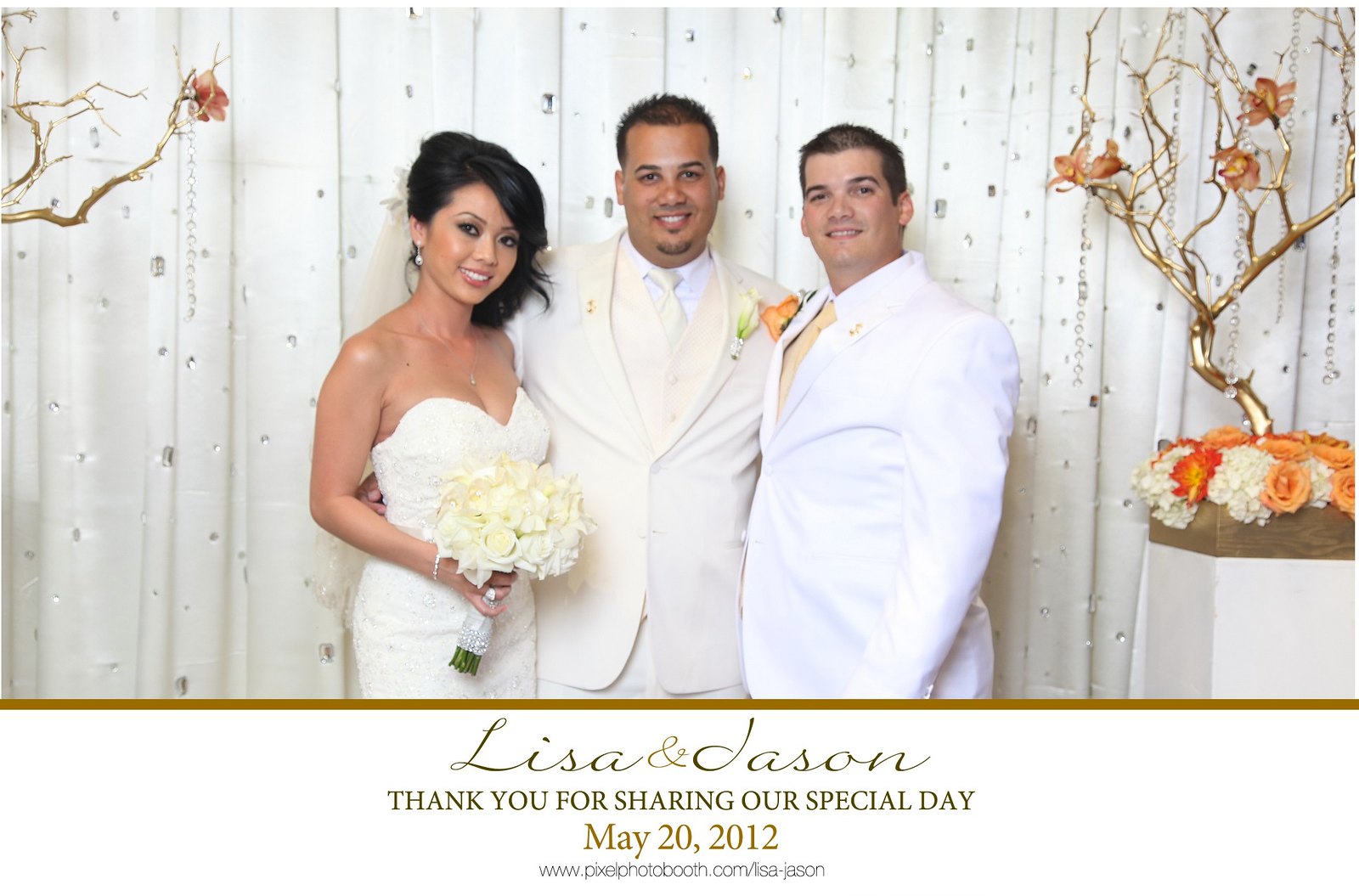The image captures a heartfelt moment from a wedding, prominently featuring a "Thank You" card at the top. It shows three people standing in front of an ornate white curtain adorned with gemstones and branches that appear to have been spray-painted gold. On the left, a woman, presumably Lisa, is dressed in a strapless wedding gown and is holding a white bouquet. She is accessorized with dangling earrings, a plunging necklace, and has her hair styled in a classic bridal fashion, swept to the side. Central to the photograph is a man in a cream-colored suit with a matching tie and a white shirt, likely Jason. To the right, another man is dressed in a white suit with a cream-colored tie and an orange flower in the pocket. The background is decorated with a shimmering white backdrop and white, orange, and yellow flowers. Below the photo, the text reads: "Lisa and Jason. Thank you for sharing our special day. May 20, 2012," followed by a link to pixelphotobooth.com/Lisa-Jason.